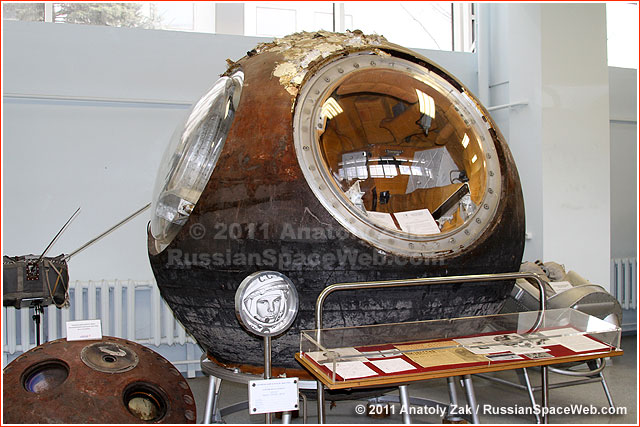This photograph depicts an aging, spherical Russian space capsule prominently displayed in a museum setting. The capsule's exterior is dark red and black, marred with burn marks, suggesting re-entry into Earth's atmosphere. It features large, clear glass openings resembling bubbles, providing a glimpse into its yellow interior. In front of the capsule, a small podium bears the outline of an astronaut's face. Adjacent to this podium is a long rectangular table covered with glass, which houses documents and photographs related to the capsule. The museum display also includes various space-related artifacts, including another rusted, glass-paneled object and a gray contraption. The scene is lit by windows at the top of the white room, which also features radiators against the back wall, adding to the historical ambiance of the exhibit.